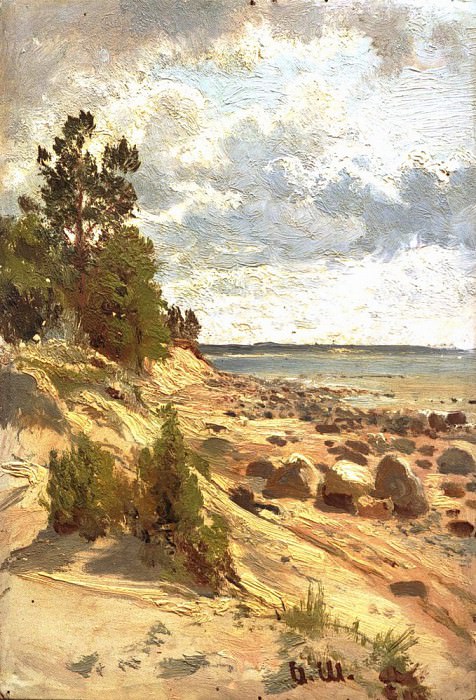The painting is a detailed oil depiction of a rocky, sandy beach, likely at the edge of a lake or bay, given the lack of waves and exposed rocks suggesting low tide. The sky is a dramatic blend of white, blue, and gray, with swirling clouds that show light and dark patches, perhaps hinting at an impending rain. The foreground showcases a scrubby, rocky stretch of sand populated with large stones. To the left, the sand rises into a small hill adorned with scattered clumps of green trees. A dense cluster of trees occupies the upper left area, while the right side features a gradient of sand dotted with small green bushes descending towards the water. The background reveals a gray expanse of water and a distant strip of darker land, creating a complex interplay of neutral colors like dark green, beige, white, and hints of orange in the sand. The texture and thickness of the oil paint add depth to this effectively crude yet evocative landscape scene.